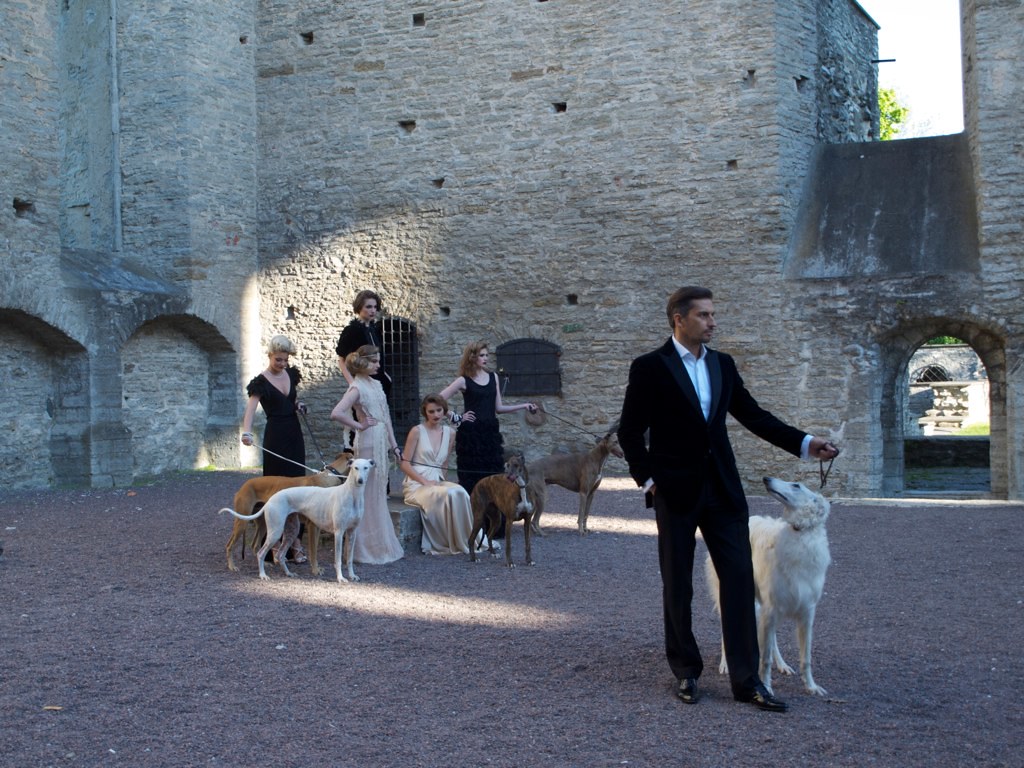The image depicts a scene of an apparent photo shoot set in a courtyard, possibly that of an old, high-stone castle with discolored walls and distinctive arched walkways. The courtyard features a brick pavement extending to a white brick wall with a door and an archway visible on the right-hand side. 

In the foreground, slightly to the right, stands a man impeccably dressed in a black suit, a white shirt with no tie, and shiny black dress shoes. His dark hair is slicked back, and he holds a white Afghan hound, a tall dog that reaches his waist, on a leash. The dog gazes up at him.

Behind the man is a small group of five women, all elegantly attired in various evening gowns that evoke a 1920s aesthetic. Three women wear black gowns, while two are in white. Four of the women remain standing as one sits. Each of the women holds a leashed dog, which appear to be greyhounds or whippets, adding a cohesive element to the sophisticated and somewhat nostalgic atmosphere of the scene.